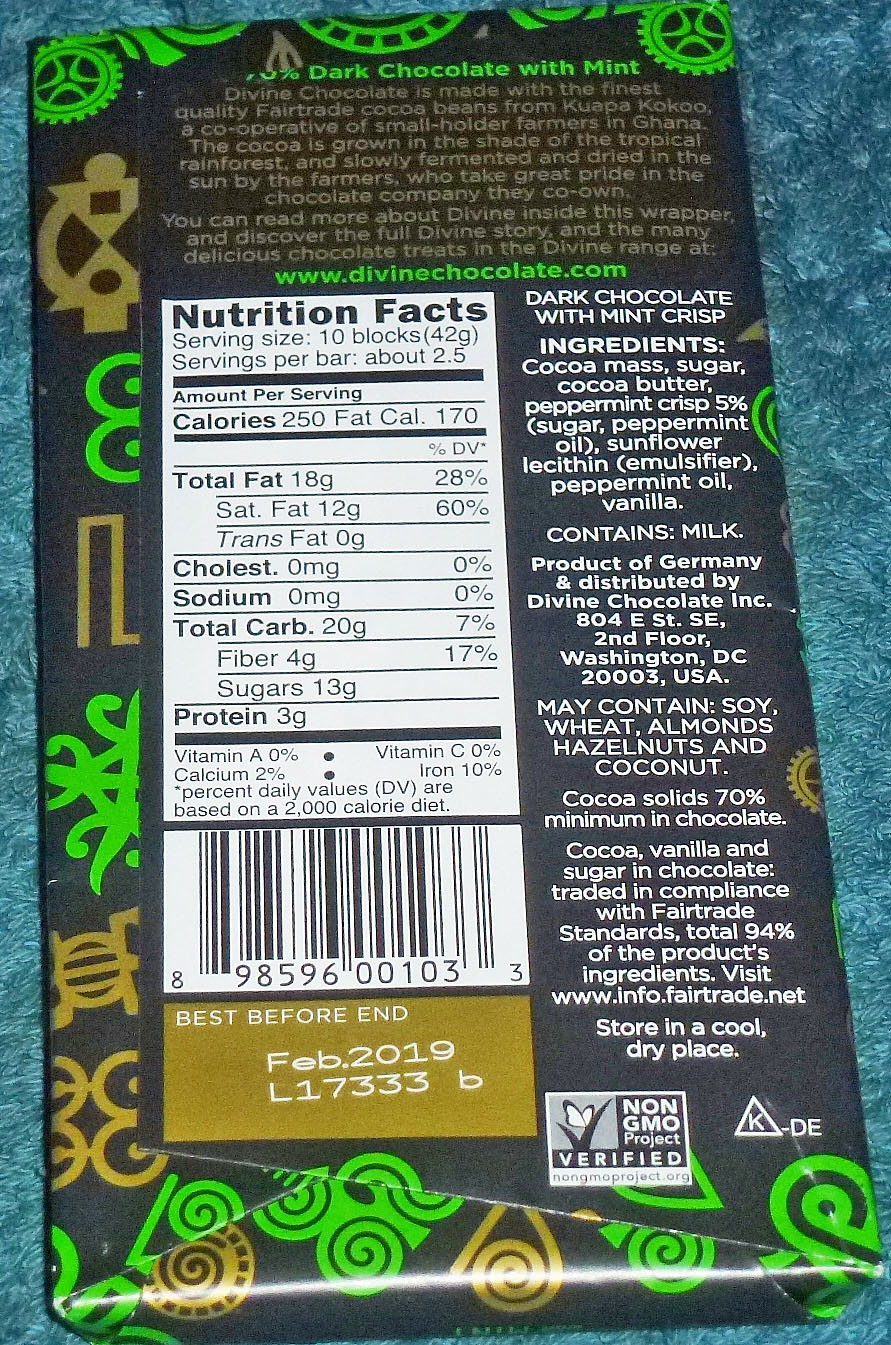This detailed photograph captures the backside of a label from a 70% dark chocolate with mint bar, a product of Germany. The label prominently features a white section detailing the nutrition facts, which include: 250 calories, 18 grams of total fat, 20 grams of total carbohydrates, 4 grams of fiber, 13 grams of sugars, and 3 grams of protein. The black label itself is intricately adorned with bright green symbols that resemble gears and Asian characters, interspersed with various gold designs, adding an elegant and exotic flair to the packaging.